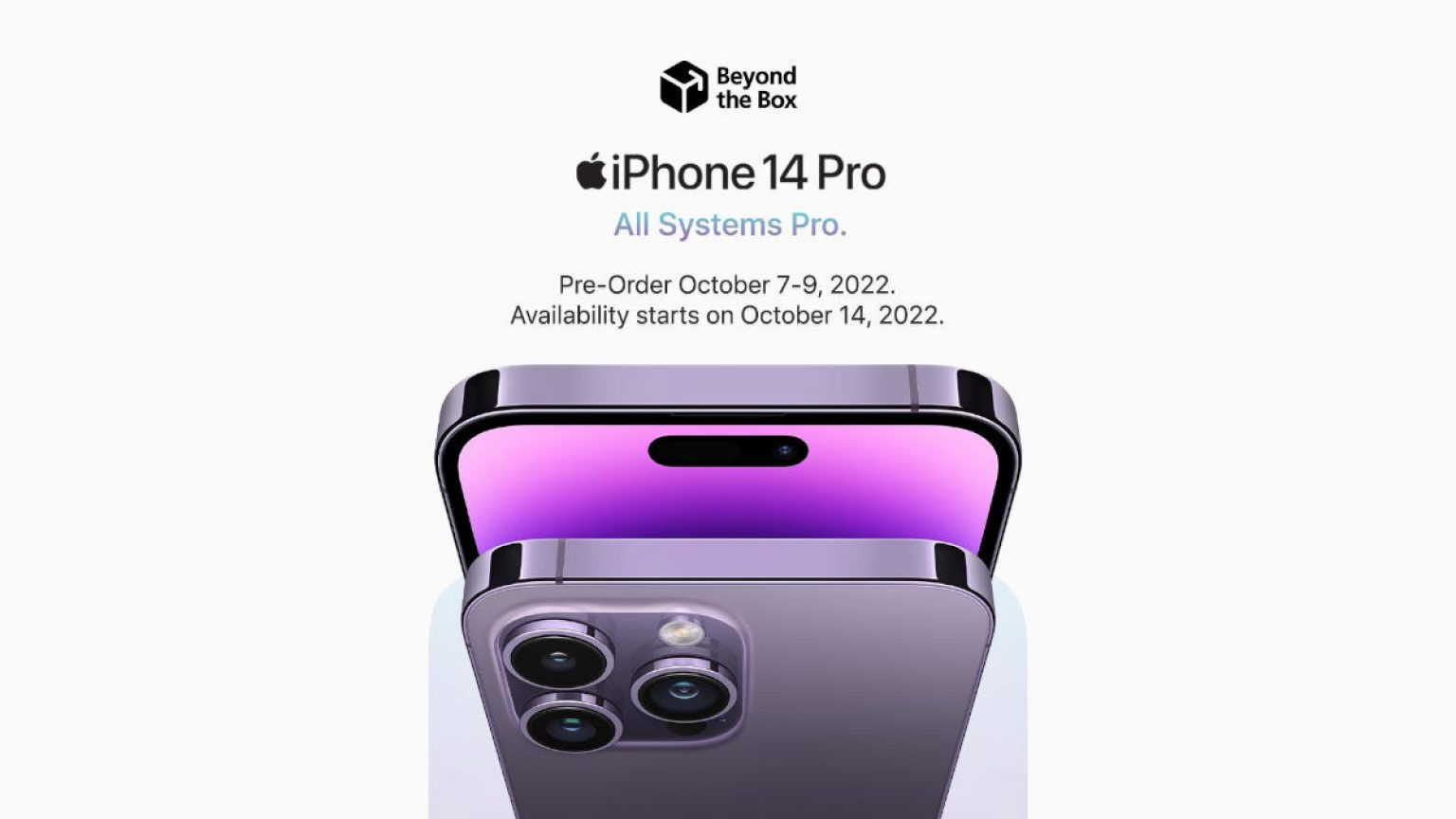This photo showcases the new iPhone 14 Pro, scheduled for pre-order from October 7th to October 9th, 2022, with availability starting on October 14th, 2022. The device is marketed by Beyond the Box with the slogan "All Systems Pro" prominently displayed in blue text. The iPhone 14 Pro is depicted in a striking gradient color scheme, transitioning from a hot pink at the center to a lighter pink towards the corners, complemented by a very shiny edge.

In the foreground, the front side of the phone is visible, highlighting its advanced triple-camera system with three round lenses. The back of the phone, shown in a light gray color with an equally shiny border, adds to the sleek and modern aesthetic. The product is centrally positioned on the page, framed by a clean white background that extends through the text description, maintaining a minimalistic and focused presentation.